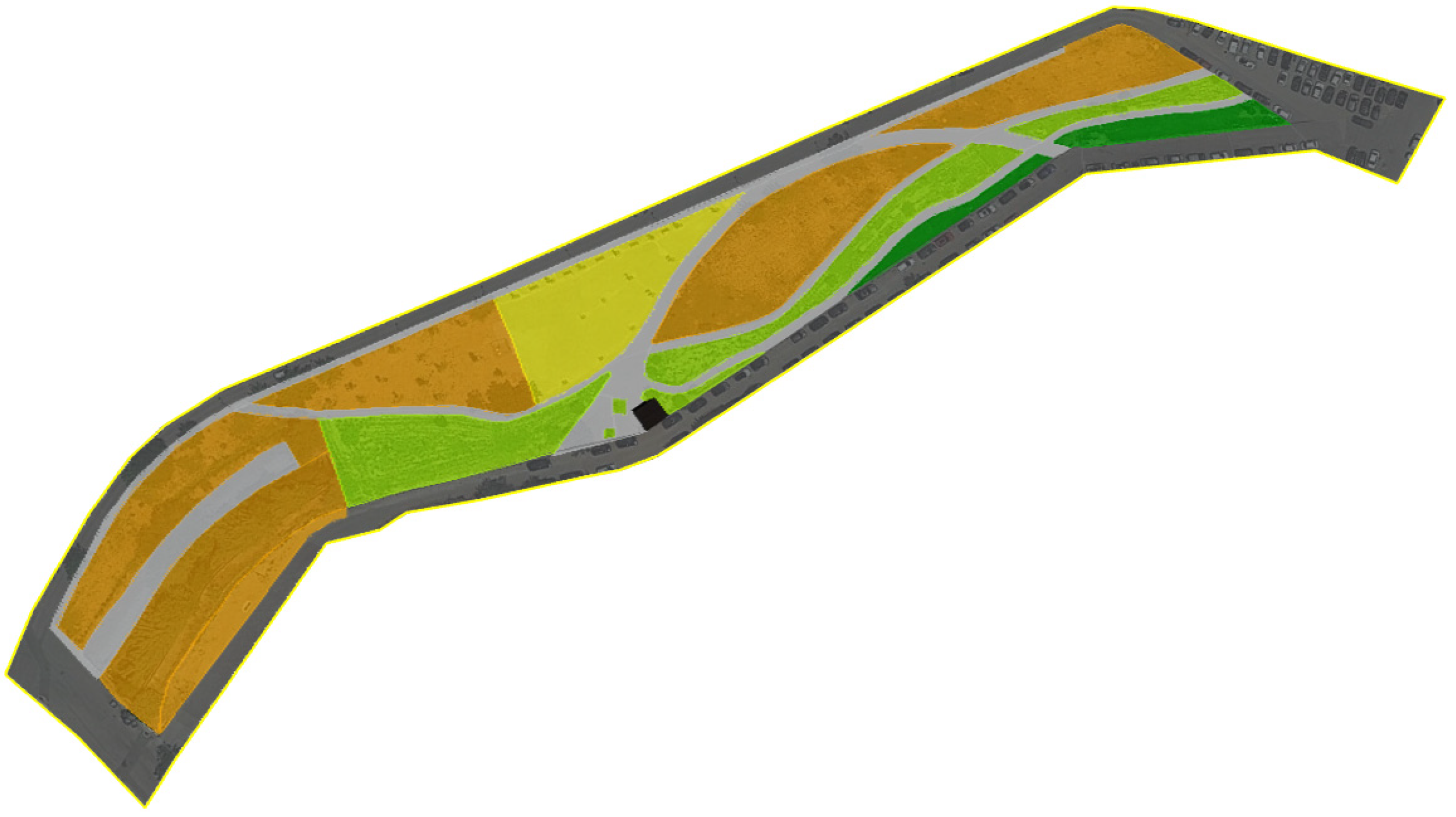This image features an intricate, hand-drawn design or possibly a plot of land, depicted with a blend of oranges, greens, and yellows. It incorporates gray lines resembling roads that traverse the image from the lower left to the upper right. The overall shape is reminiscent of a long, bent rectangle, potentially resembling an aerial view of a parking lot or map. Each section—orange, green, and yellow—is distinctly marked and bordered, creating a detailed, almost map-like illustration or design. The gray lines intersect the vibrant sections, adding a structured, road-like quality to the image.